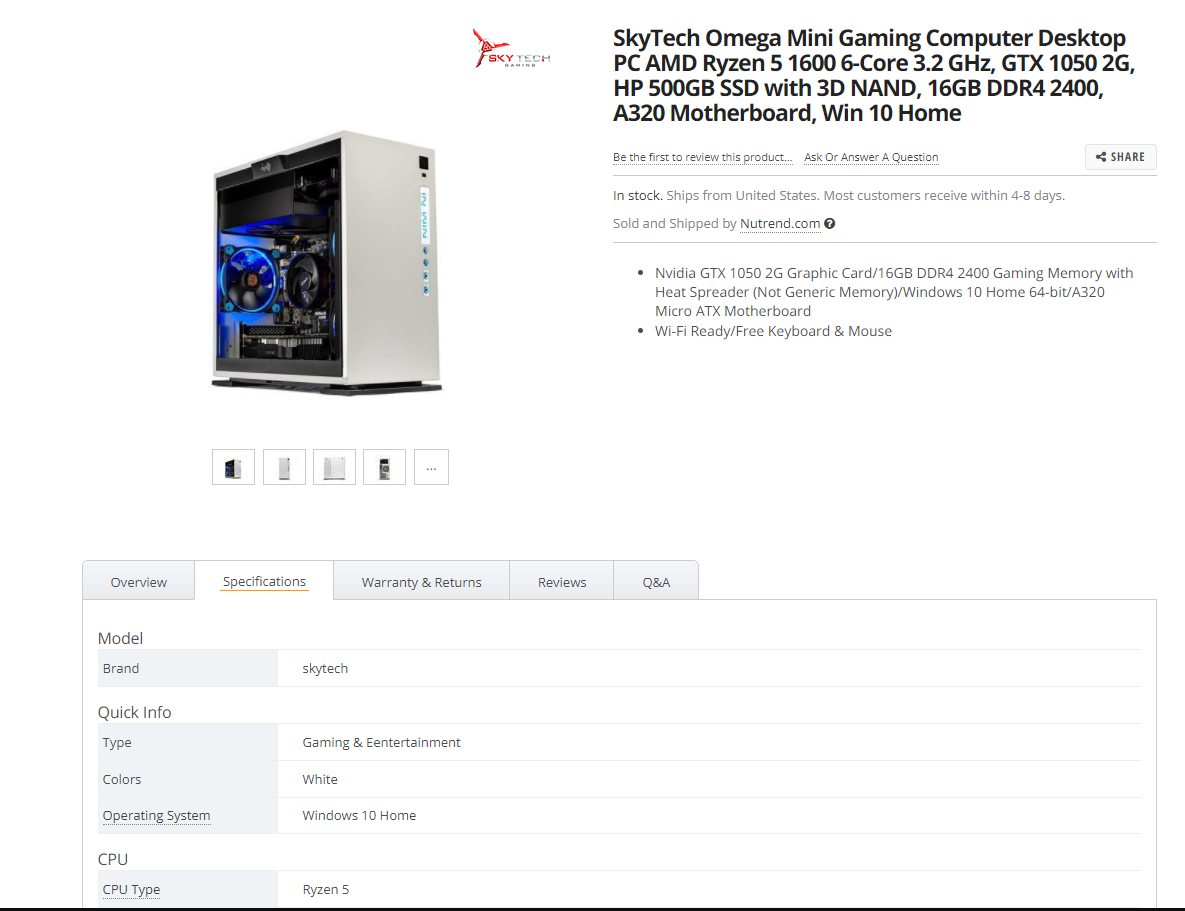**Product Overview: Skytech Omega Mini Gaming Computer**

The image depicts a detailed layout of a Skytech Omega Mini Gaming Computer on an app interface against a clean white background. Positioned one inch from the left and top edges, an open desktop computer is showcased, revealing its internal components. The computer's exterior is gray on the right side, and its interior displays a striking contrast with blue components on the left section and black components on the right section. Beneath this central image, there are four clickable thumbnails, each framed by a black border.

To the upper right of the main image, a red icon resembling a fidget spinner is displayed, with the text "Sky" in red and "Tech" in black beneath it. Adjacent to this logo, bold black lettering provides a detailed product title and specifications across four lines:

- Skytech Omega Mini Gaming Computer Desktop PC
- AMD Ryzen 5 1600 6-core 3.2 GHz
- GTX 1050 2GB GPU
- 500 GB SSD with 3D NAND, 16 GB DDR4 2400 MHz RAM
- B320 motherboard, Windows 10 Home

Below this descriptive text, there are two clickable tabs with black lettering. On the right side, a gray "Share" tab with a share icon is also visible. Beneath this, further information is arranged with two more lines, indicated by dots on the left side. The top dot signifies three lines of data, while the bottom dot contains one line.

In the lower-left section, a gray "Overview" tab is present, with a black label. Adjacent to this, a white "Specifications" tab, underlined in yellow, stands out. Additional tabs titled "Warranty and Returns," "Reviews," and "Q&A" follow in black lettering.

On the right side, product details continue with sections labeled "Model" and "Brand," where "Skytech" is highlighted in a blue tab within a white rectangle spanning the width of the layout. Below this, "Quick Info" is sectioned with a blue background, listing information from top to bottom as "Type," "Colors," and "Operating System," with "Gaming," "Entertainment," "Windows 10 Home," and "CPU" details respectively.

Overall, the image offers a comprehensive and visually organized view of the Skytech Omega Mini Gaming Computer's features and specifications.